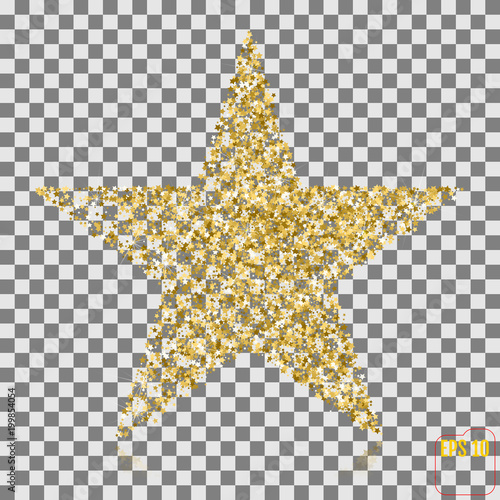The image features a prominent, five-pointed star situated in the center of a square background. The star, made of gold glitter with colors ranging from light gold to dark brown, appears semi-transparent, allowing the checkerboard pattern background to show through. The background itself consists of alternating white and dark gray squares, creating a striking contrast with the glittery star. The star's points extend upward, to the left, to the right, and both lower corners. In the lower left-hand corner of the image, "Adobe Stock" is printed vertically, followed by an unreadable number. The lower right-hand corner features a small red circle enclosing the text "EPS10" in yellow font.